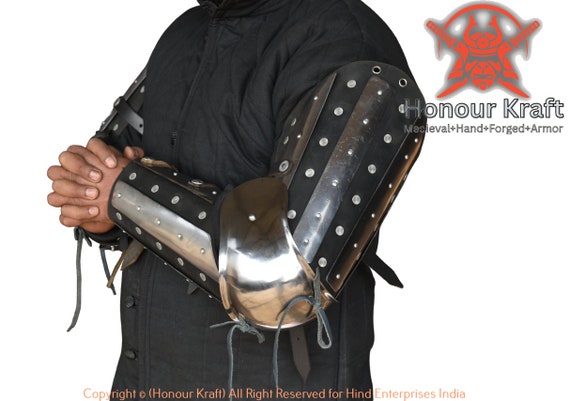The image features a close-up of a person, possibly male, whose head is not visible, dressed in a black, Renaissance-style jacket with armor that extends from their shoulders down to their wrists on both arms. The metal armor is intricately detailed with silver metallic dots and circles, held together by strings and fastenings. Both hands are clasped together in front of the torso, and the individual is turned slightly to the left. 

The background is plain white, emphasizing the armor and attire. In the top right corner, there is a red logo depicting a samurai face with crossed swords behind it, accompanied by the text "Honorcraft Medieval Hand Forged Armor." The bottom left corner features a copyright notice: "Copyright Honorcraft All Rights Reserved for Hind Enterprises India." This image serves as an advertisement for the company's handcrafted armor.